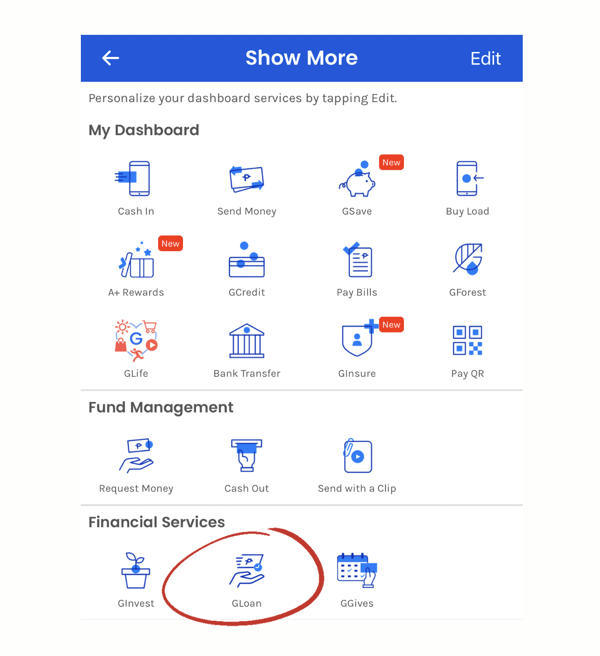The image is a screen capture of a digital menu interface, which could be from either a mobile device or desktop. At the top of the screen, there is a header with a "Show More" option. This is followed by a menu row that features a back arrow on the left and an "Edit" button on the right, indicating that the menu can be customized. Directly below this row, there is instructional text that reads, "Personalize your dashboard and services by tapping edit."

The main content area is titled "My Dashboard." Below this title, there is a grid comprised of 12 icons, arranged in a 4x3 layout, spread across three rows. The icons and their labels are as follows:
- First row: Cash In, Send Money, G-Save, Buy Load
- Second row: A+ Rewards, G-Credit, Pay Bills, G-Forest
- Third row: G-Life, Bank Transfer, G-Insure, Pay QR

A horizontal dividing line separates "My Dashboard" from the section below, titled "Fund Management." This section contains a single row with three icons labeled: Request Money, Cash Out, Send with Clip.

Another horizontal line divides this section from the final section titled "Financial Services." This last section features three icons in a row labeled: G-Invest, G-Loan, and G-Gives. Notably, the G-Loan icon and its label are highlighted with a red circle.